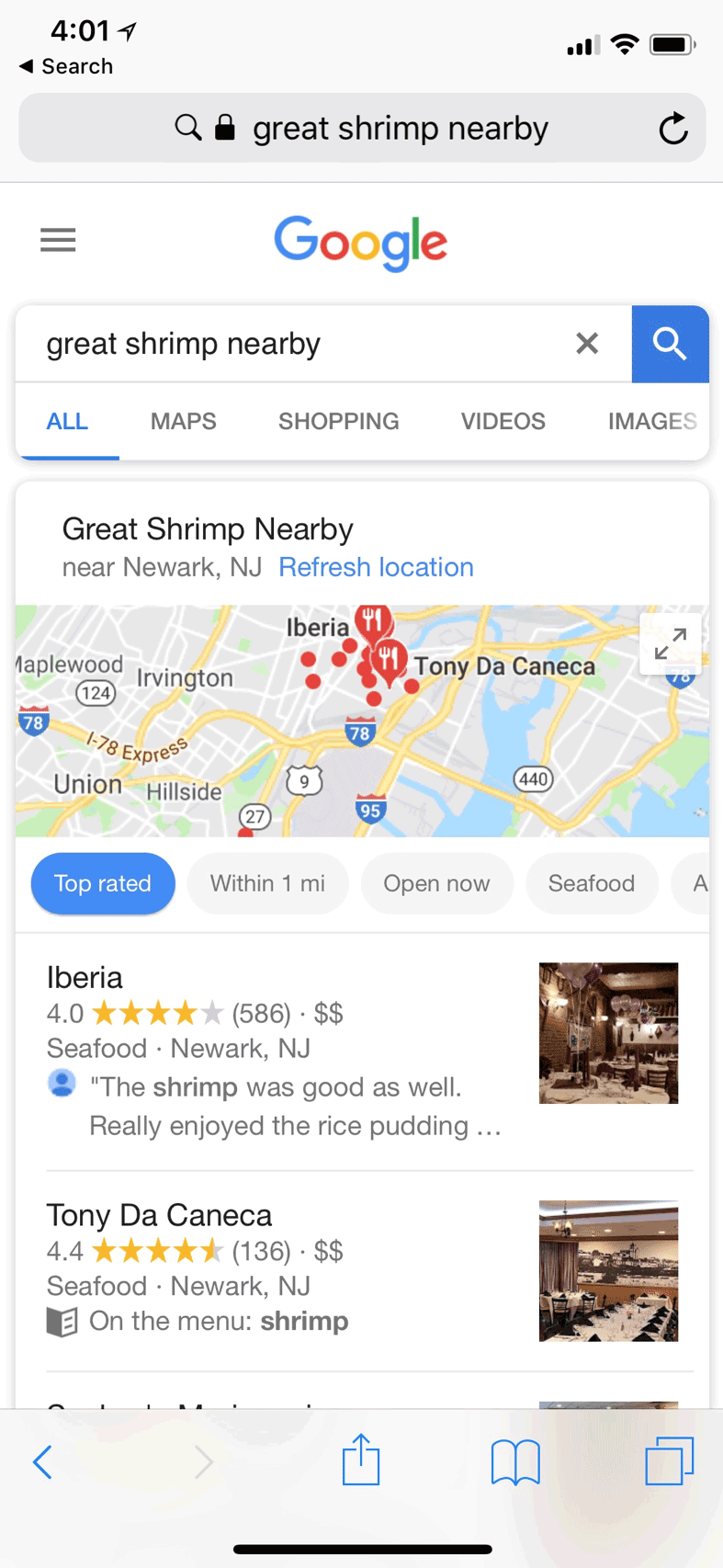The screenshot captures a mobile device displaying a Google search interface with a clean light gray background. At the top-left corner, the time "4:01" is shown, while the top-right corner indicates the battery status, Wi-Fi signal, and cellular signal strength icons. Below the time, a search bar features a left-pointing arrow, a magnifying glass icon, a padlock icon, and the text "great shrimp nearby." Beneath the search bar, on a white background, the prominent "Google" logo is presented beside the repeated search term "great shrimp nearby," accompanied by a close (X) icon and a blue square housing another magnifying glass icon, symbolizing the search action.

Further below, there are navigational options labeled "All," "Maps," "Shopping," "Video," and "Images," with "All" highlighted in blue and underlined, signifying it as the current selection. The text "great shrimp nearby near Newark New Jersey," is displayed with "refresh location" in blue, suggesting it is an actionable link. The screenshot then shows a map of Newark, NJ, dotted with red markers, representing various seafood restaurants—all marked with a fork and knife icon. At the bottom of the screen, there's a list headed "Top rated within one mile - open now: seafood," including listings for "Iberia," "Tony" and partially cut-off text possibly reading "CONNECT USA" with capital letters "D," "C," and "ECA," indicating further details about the establishments.